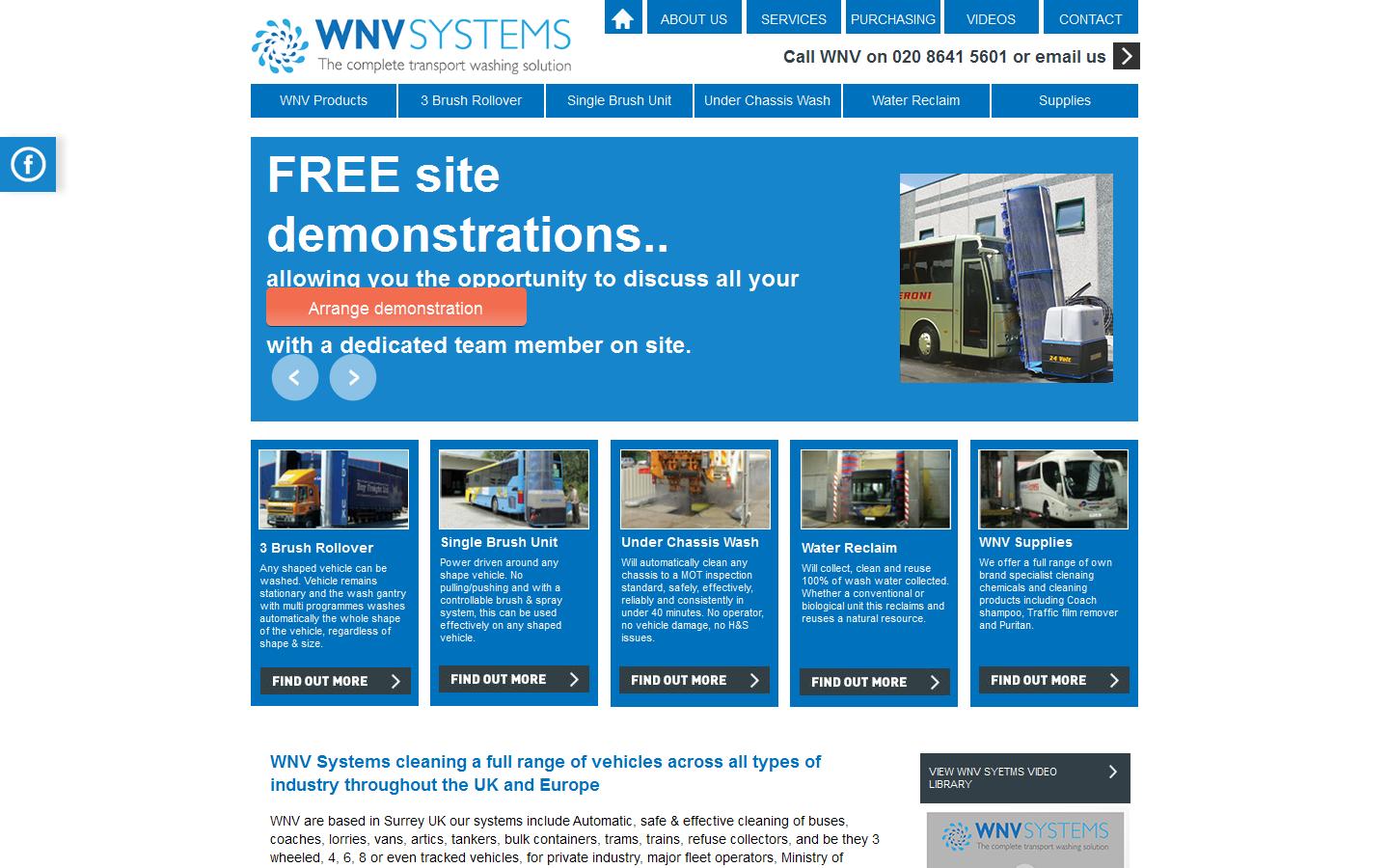The screenshot showcases the homepage of the WNB Systems website. The branding, 'WNB Systems,' appears prominently on the left side in bold blue text accompanied by a circular logo made of small dots and waves.

At the top of the page, there is a navigation menu with blue buttons annotated as Home, About Us, Services, Purchasing, Videos, and Contact. Additionally, there's a prominent call-to-action section urging users to "Call WNB on 020 8641 5001 or email us," flanked by a black arrow pointing right, and a button labeled "Why Products?"

The central part of the page features a large, bold headline in white text: "Free Site Demonstrations" followed by a prompt inviting potential clients to "Arrange a demonstration with a dedicated team member on-site." This section includes clickable elements: an orange button for scheduling a demonstration and two additional buttons, one showcasing a bus and another with an image obscured by a box with a black base.

Below this section, there are five images depicting the equipment and services that WNB Systems uses for site and vehicle demolition. A blue footer text reads, "WNB Systems: Cleaning a full range of vehicles across all types of industry throughout the UK and Europe," suggesting their specialization in vehicle cleaning services, including buses.